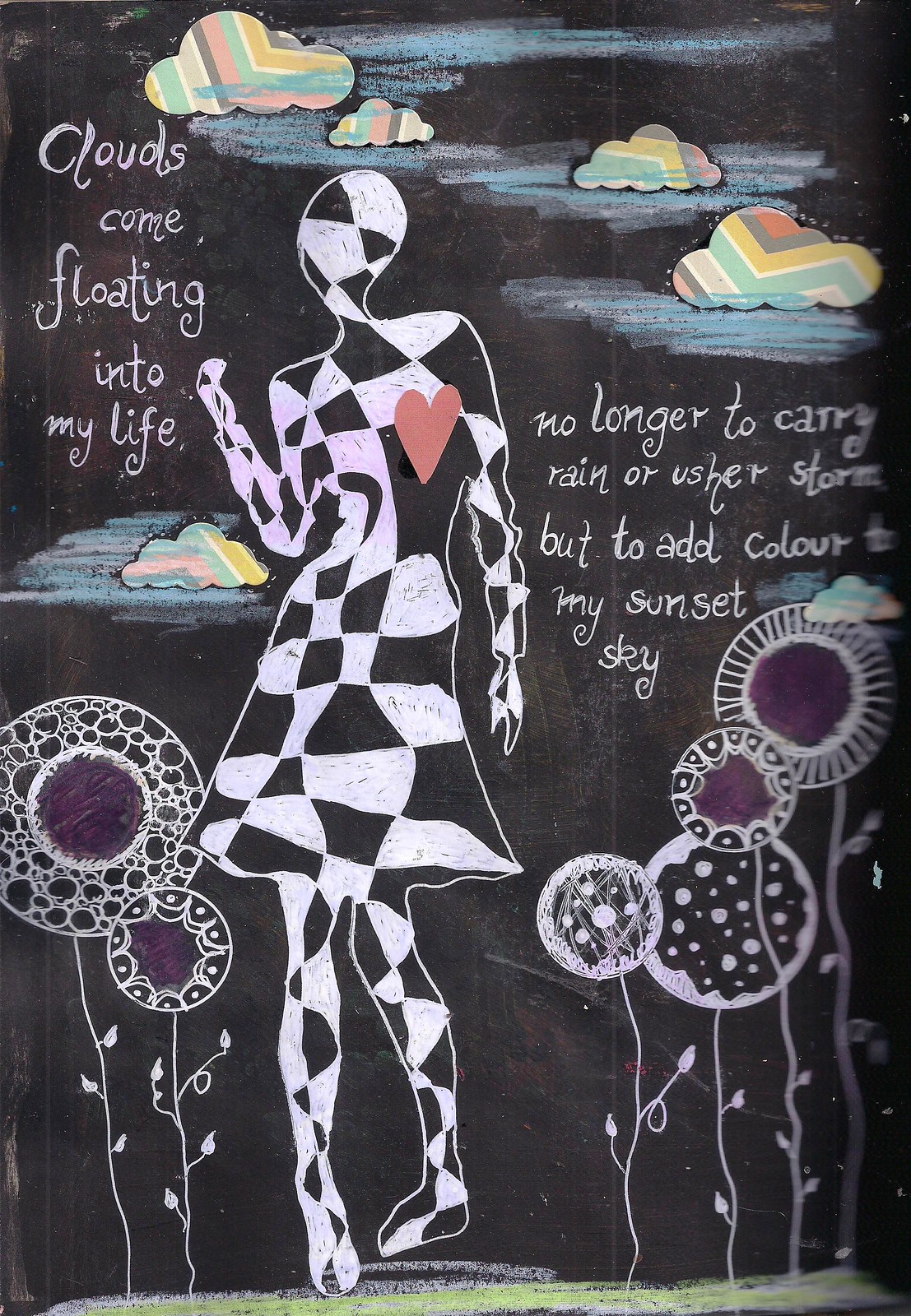This artistic image, possibly crafted on a black chalkboard, features a central figure of a woman adorned in a dress, her form sculpted with a distinctive black and white checkered pattern that encompasses her entire body, including her face. A bright pink heart is prominently placed on the left side of her chest. The background is adorned with muted primary-colored clouds, resembling a rainbow in shades of pink, brown, white, and yellow, creating a dreamlike atmosphere. Rising from the ground are abstract, round balloon-like flowers depicted in black and white, with hints of purple chalk at their centers. Surrounding the woman on both sides is a beautifully inscribed poem: on the left, "clouds come floating into my life," and on the right, "no longer to carry rain or usher storm, but to add color to my sunset sky." This imaginative piece blends elements of chalk art with poetic words to create a visually and emotionally captivating scene.